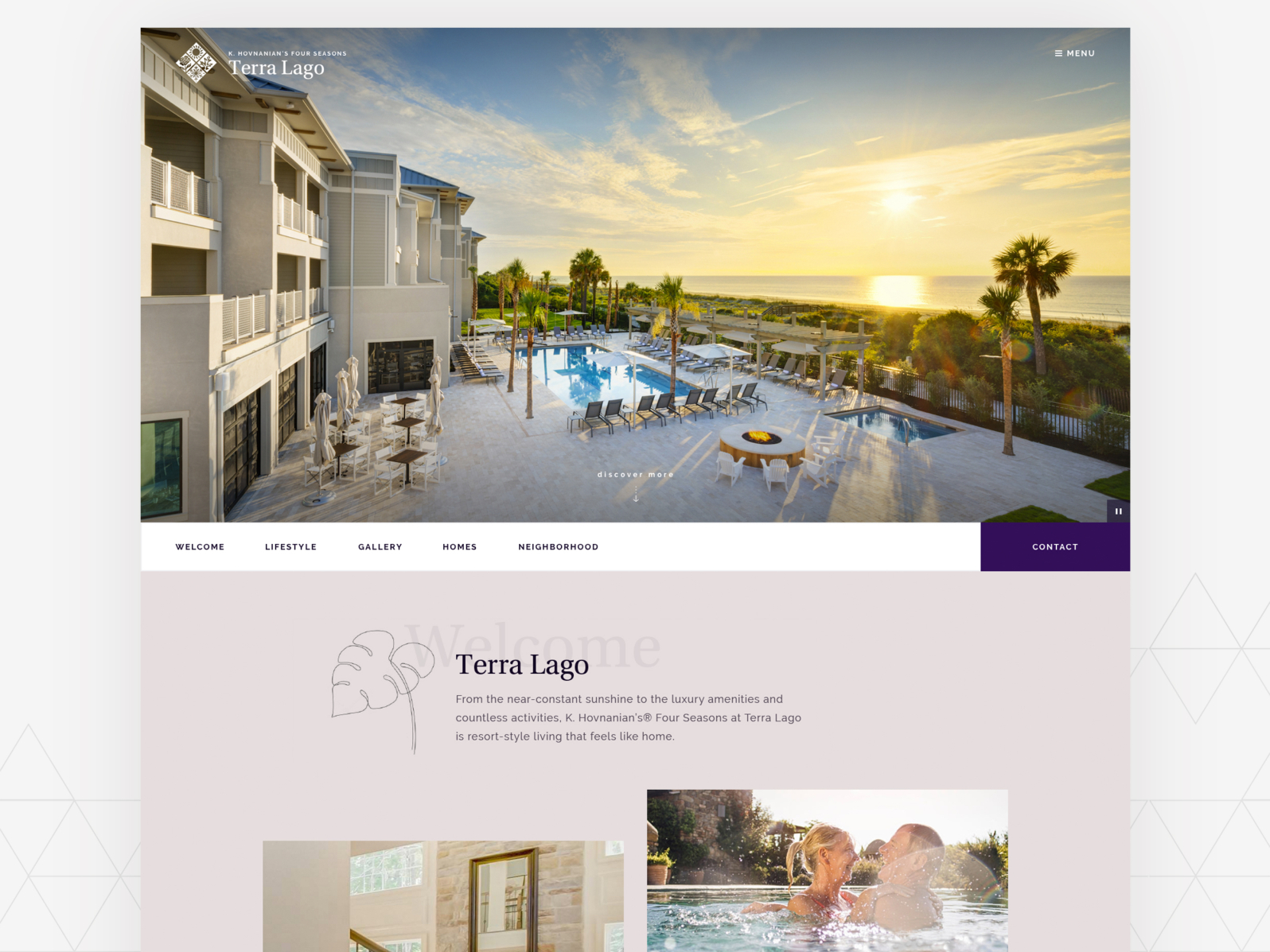A vivid screenshot depicts a serene sky with scattered clouds and radiant sunshine reflecting off calm water. In the right corner, a navigation menu is visible, featuring options: "Welcome," "Lifestyle," "Gallery," "Homes," "Neighborhood," and "Contact," all in white text against a purple background. The setting appears to be Terra Lego, with luxurious apartment buildings that resemble a high-end hotel. The complex boasts a swimming pool, lush palm trees, and a pristine white picket fence. With near-constant sunshine, Terra Lego offers resort-style living with an array of amenities and activities to enjoy. Accompanying the main image are two inset pictures: one showing an elegant interior of a home, and the other capturing a couple enjoying time together in the pool.